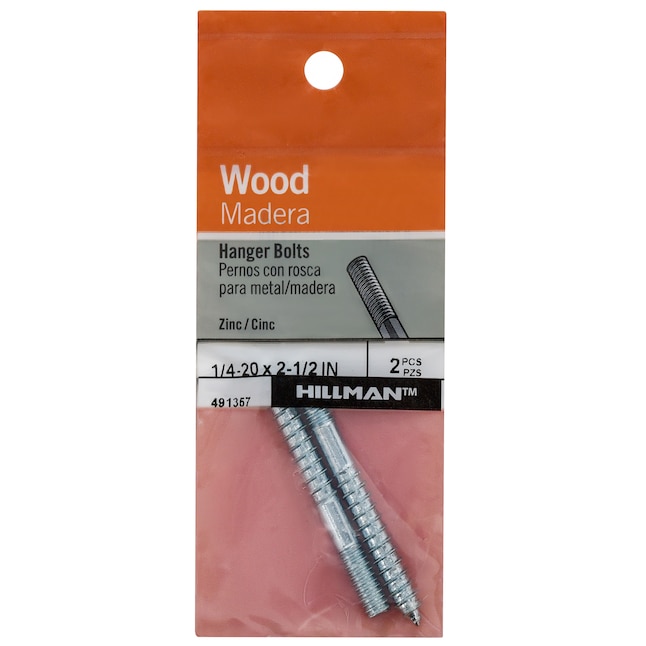This photograph depicts a rectangular package containing two zinc hanger bolts, clearly visible through a transparent plastic section set against an orange background. The top of the package features a large orange square with a hole punched for hanging on a rack. Below the hole, the brand name 'Wood Madeira' is prominently displayed in white letters. Beneath this, a gray strip bears the term 'Hanger Bolts' in bold black letters, with further information and a picture of the bolts provided below in another language. The bolts themselves look like large screws and are shiny silver. Measurements are noted in black letters as 1/4"-20 x 2 1/2", indicating the size and gauge of the bolts. It is suggested that Wood Madeira is the marketer, while the actual manufacturer might be Hillman, as indicated by a trademark on the packaging.